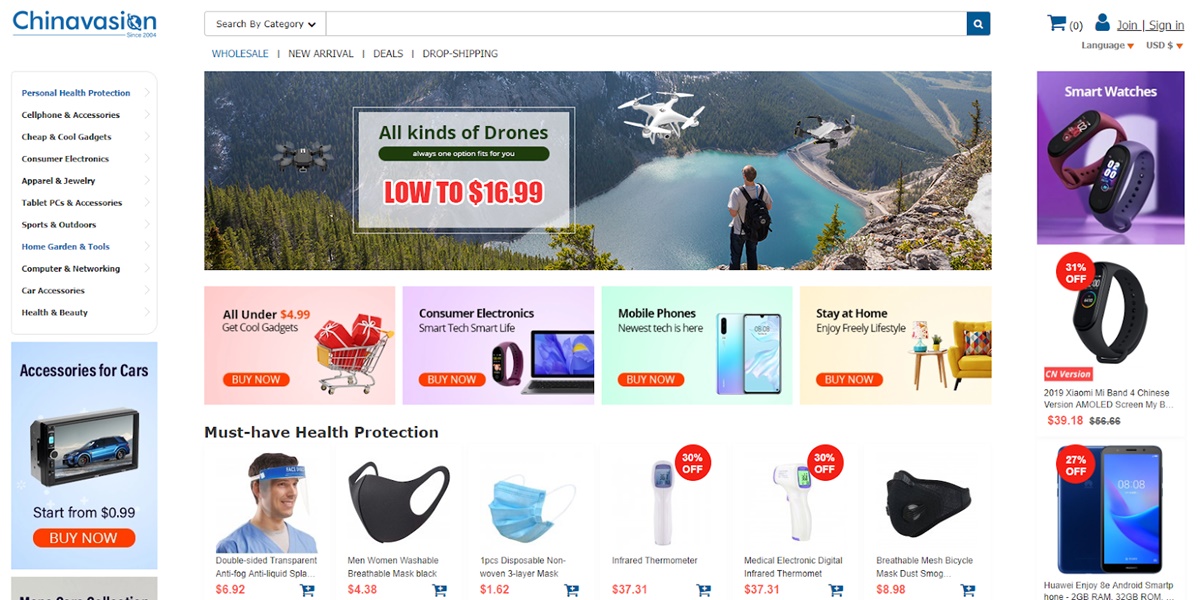This image depicts a meticulously designed sales page from the e-commerce website China Vision, established in 2004. The webpage is organized with various shopping categories prominently displayed, including: 

- Wholesale
- New Arrivals
- Deals
- Dropshipping 
- Personal Health Protection
- Cell Phones & Accessories
- Cheap and Cool Gadgets
- Consumer Electronics
- Apparel and Jewelry
- Tablet PCs & Accessories
- Sports and Outdoors
- Home, Gardening, and Tools
- Computer and Networking
- Car Accessories
- Health and Beauty

On the left-hand side, there are quick links for easy navigation. Further down the page, featured sections include must-have health protection items such as double-sided transparent, anti-fog, anti-liquid masks which are washable and breathable, available in black, blue, red, and brown. Additional offerings include affordable car accessories starting at $0.99, as well as an assortment of trending gadgets like drones, smart watches, and Fitbits. The layout is user-friendly and visually appealing, catering to a wide range of consumer needs.